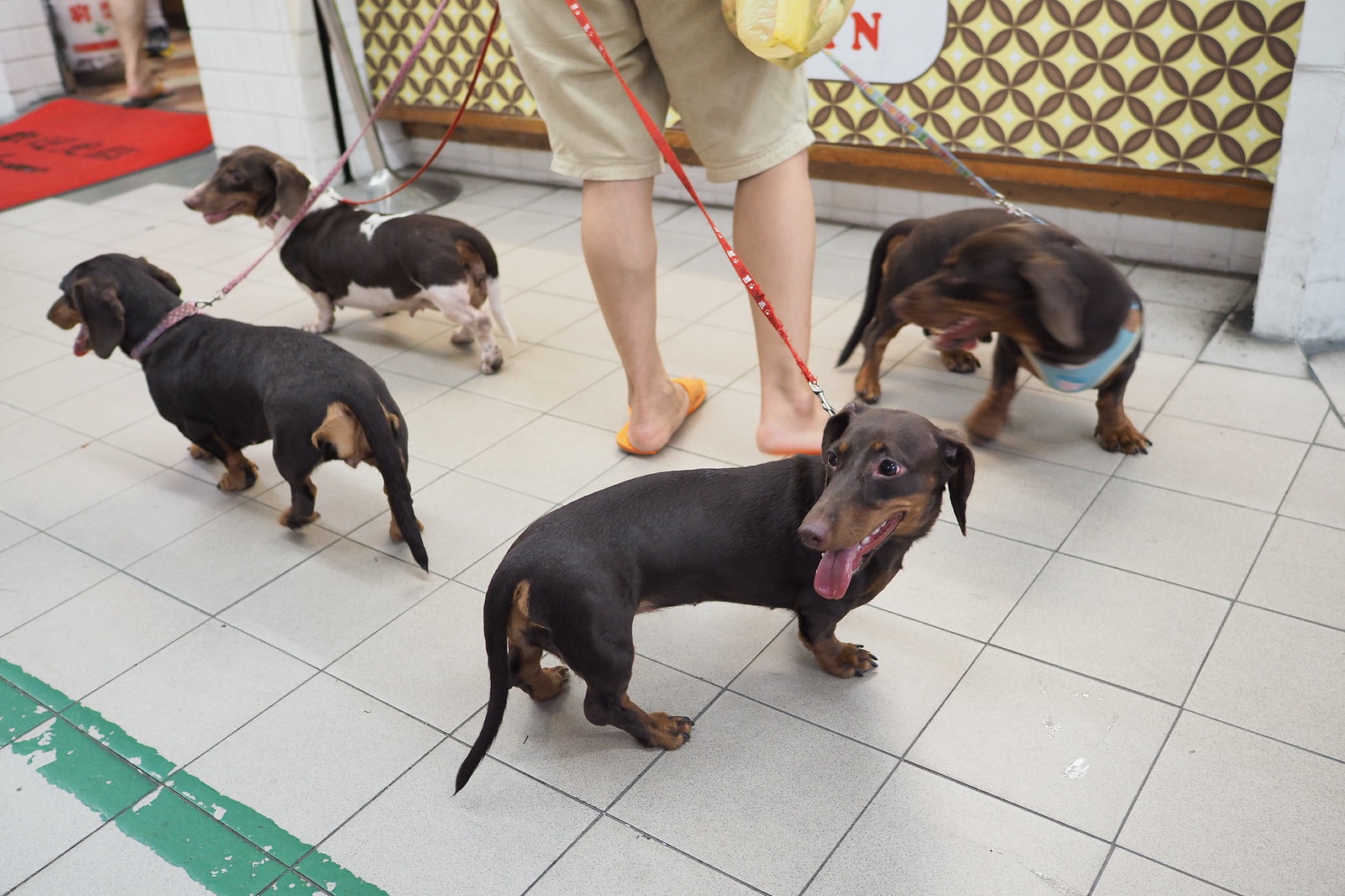A person wearing yellow flip-flops and light brown shorts is standing on a tiled floor, holding the leashes of four small, brown dogs with black and white accents. The leashes are of various colors: two red, one purple, and one gray. The dogs, which appear to be wiener dogs, are facing different directions, with one turning and smiling with its tongue out. The person is standing in front of a wall that features a sign they are reading, with circles of brown and a yellow star pattern on it. The scene is set in what might be a subway or the entrance of a small business, indicated by a red carpet with advertising in the background and an opening leading further inside. The tiled floor beneath them is predominantly white with streaks of green. Other people can be seen in the background, suggesting a public or semi-public location.